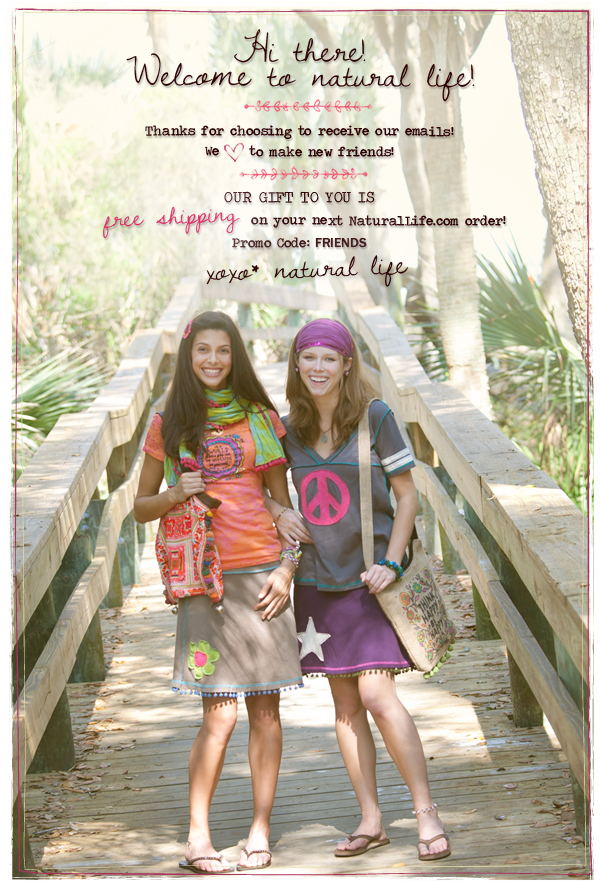In the image, two young women are standing closely together on a pedestrian wooden bridge, which is surrounded by lush tropical trees. Both women are smiling brightly and appear to be enjoying the moment as they pose for the camera.

The woman on the right is dressed in a coral-colored t-shirt with a circular design, paired with a skirt that features an embroidered flower. She accessorizes with a scarf wrapped around her neck, a purse on her shoulder, and thong sandals. Her long dark hair cascades down, complementing her warm smile.

The woman on the left also sports a vibrant outfit, consisting of a v-neck t-shirt with a peace sign on the front, and a skirt adorned with little ball fringe and a star applique. She wears a purple scarf over her long, shoulder-length hair, and carries a bag similar to her companion's. Like the woman on the right, she is also wearing thong sandals and smiles brightly at the camera.

Both women are adorned with bracelets and appear youthful and vibrant, embodying a cheerful and relaxed atmosphere. The top of the picture features a text advertisement from the brand "Natural Life," which welcomes viewers, mentions free shipping on their next order with a promo code, and conveys a friendly message from the company.